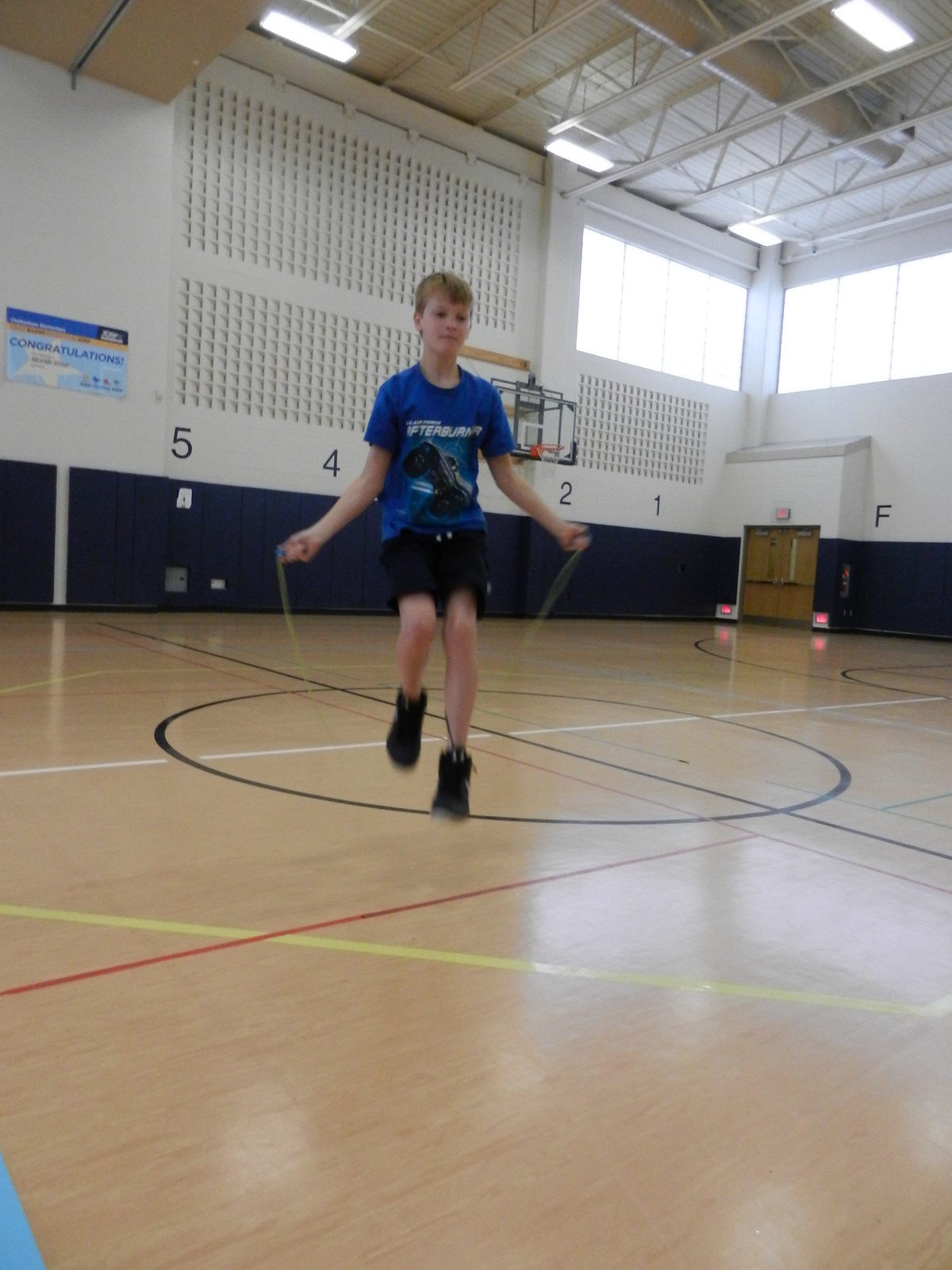A young boy with short blondish hair is captured mid-jump as he plays with a white jump rope in the center of a spacious gymnasium. The gym features a hardwood floor marked with black, red, and yellow lines for various sports, such as basketball and indoor soccer. The boy wears a blue t-shirt with a monster truck design, black shorts, and black shoes. Behind him, white walls adorned with large black numbers '5, 4, 3, 2, 1' and the letter 'F' stretch around the room. The gym's high ceiling and large windows allow ample light to flood in. Wooden doors and a basketball hoop mounted on the wall add to the gym's sporting ambiance, while additional pictures or signs are visible in the distance, though too far to discern clearly. The boy's active posture, with one leg raised and the other on the ground, showcases his joyous engagement in the activity amidst the empty, cavernous space.